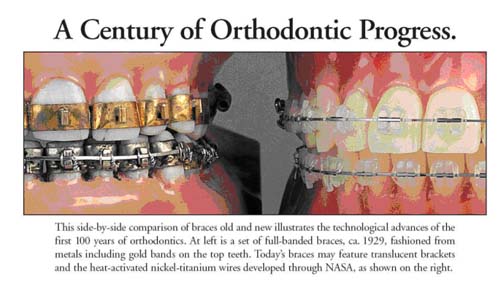The image, titled "A Century of Orthodontic Progress," is a detailed side-by-side comparison of braces from 1929 and modern times. The left half of the image features zoomed-in teeth with metallic, full banded braces, including gold bands on the top teeth, typical of circa 1929. On the right, the modern braces showcase translucent brackets and heat-activated nickel-titanium wires, innovations developed through NASA technology. The image is contained within a long, thin rectangle, presenting the teeth and orthodontic equipment in a model-like format, rather than an actual human mouth. Above the image is a headline in black text: "A Century of Orthodontic Progress," and below it, the caption explains how the comparison illustrates the significant technological advancements in orthodontics over the past 100 years.